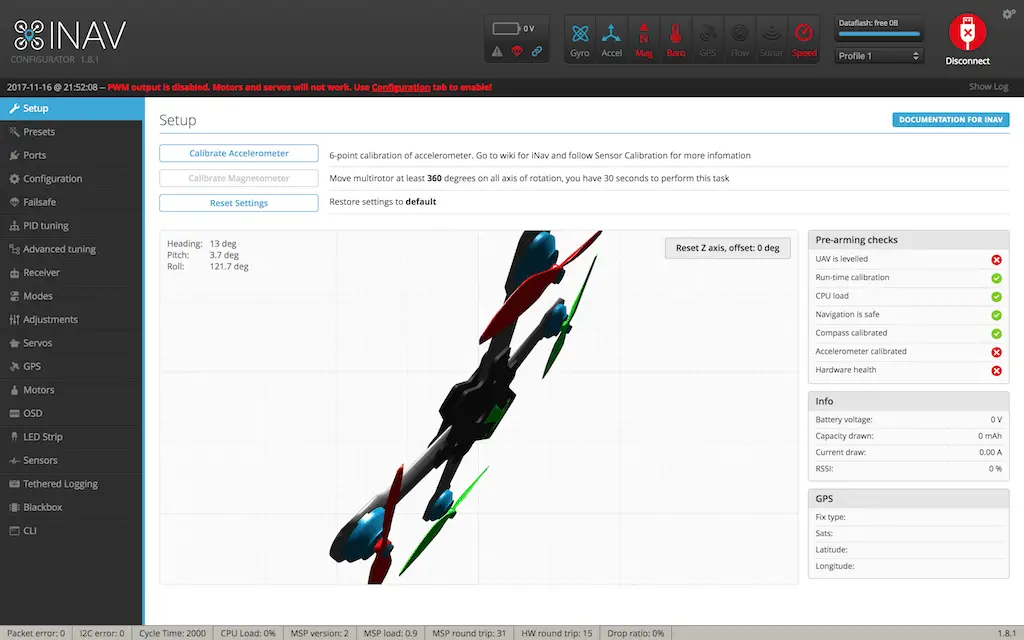This detailed caption succinctly describes a screenshot of an application interface:

"A screenshot depicts a desktop application named INAV, prominently displayed at the top left in all capital letters. Below the name, in smaller, faded text, it reads 'Configurator 1.8.1'. The logo, resembling a blue location symbol encircled by four interconnected grey circles, further brands the interface. The application's color scheme blends grey, blue, and red. 

On the left side, a pull-up menu bar lists multiple options including Setup, Presets, Ports, Configuration, Fall Safe, PID Tuning, Advanced Tuning, Receiver, Modes, Adjustments, Servos, GPS, Motors, OSD, LED Strip, Sensors, Headlight Logging, Black Box, and CLI. The active tab is 'Setup', positioned at the top of the menu.

Central to the screen is a detailed CGI representation of a drone. To the right, three informational cards are displayed, titled 'Pre-Arming Checks', 'Info', and 'GPS', each providing specific data about the drone."